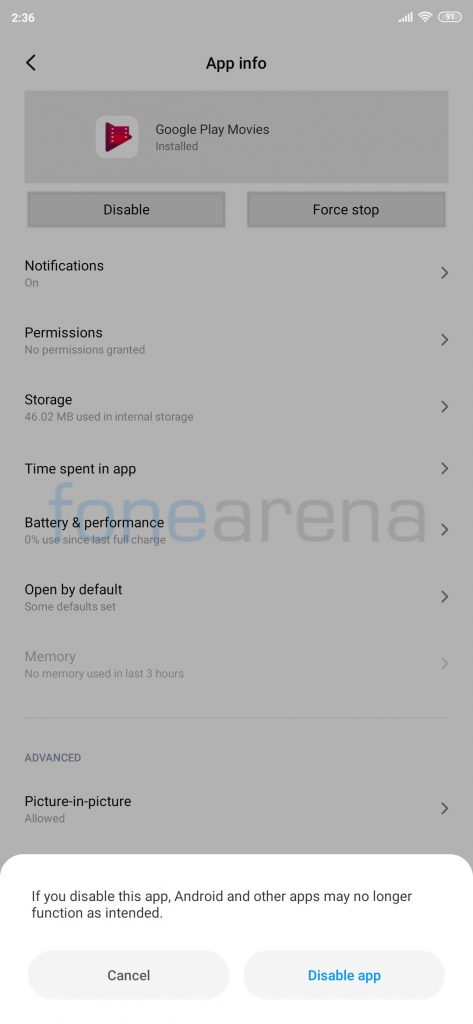The image depicts the "AppInfo" screen for Google Play Movies on an Android device. In the top left corner, "236" is displayed, indicating the app's version. The screen allows you to return to the previous menu. Dominating the center of the screen is a large gray rectangle with a red film reel logo, representing Google Play Movies, which is installed on the device.

Below the app icon, there are two rectangular buttons: "Disable" and "Force Stop". Beneath these buttons is a detailed list of options. The "Notifications" section indicates that notifications are enabled. The "Permissions" section shows that no permissions have been granted to the app. The "Storage" section details the internal storage used by the app. The "Time spent in app" section is available for viewing but currently not displayed. The "Memory and performance" section indicates 0% usage, with the device at a full charge. The "Open by default" section offers an option to open the app by default to this screen. Additionally, the memory usage section confirms that no memory has been used in the past three hours.

A slightly darker gray line separates the main options from the "Advanced" section, which includes "Picture in picture" functionality, indicating that it is allowed. At the bottom of the screen, there is a warning that disabling the app may cause Android and other apps to malfunction. Users have the option to cancel this action or confirm by tapping the blue "Disable app" button against the gray background.